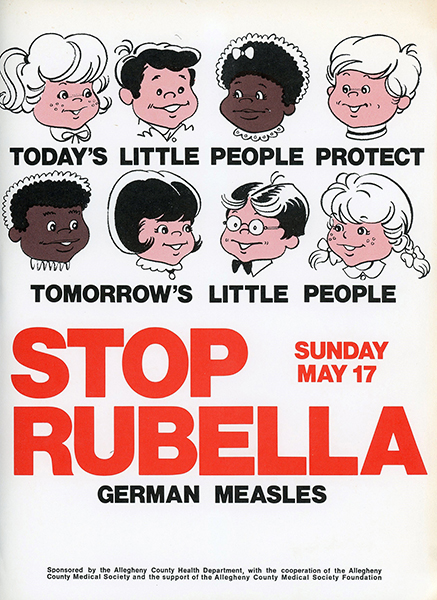This is a public service announcement poster aimed at promoting vaccination against Rubella, also known as German Measles. The poster has a white background and features eight cartoon portraits of children of various races and genders, including a black girl with an afro, a white girl with freckles and white hair, a black boy with an afro and a white stripe in his hair, and several other children with different hair and skin tones. At the top of the poster, in black font, it states, "Today's Little People Protect Tomorrow's Little People." Below the portraits, in large red font, it prominently reads, "Stop Rubella," followed by "German Measles" in smaller black font. To the side, also in red, it announces the vaccination date, "Sunday, May 17th." At the very bottom, in small black text, it credits the sponsorship and support to the Allegheny County Health Department, the Allegheny County Medical Society, and the Allegheny County Medical Society Foundation. The style and design suggest the poster likely dates from the 1970s or 1980s.